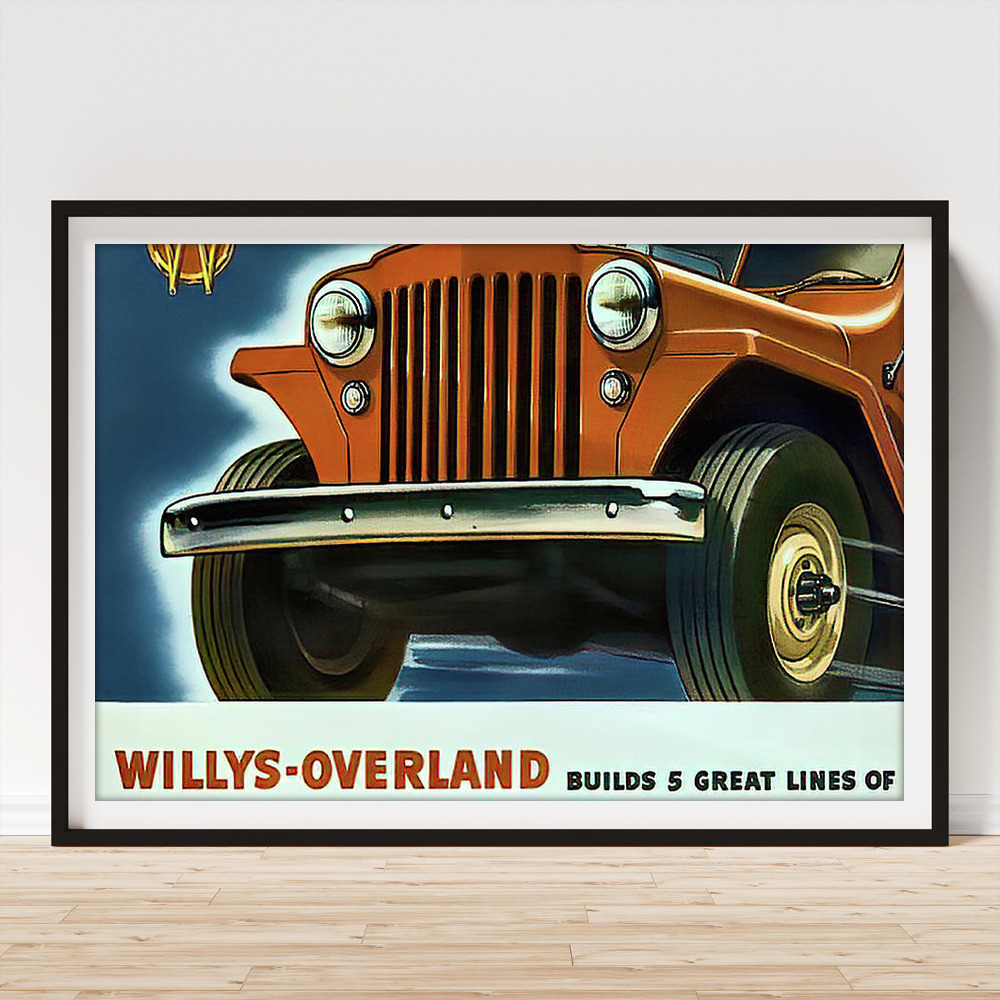The framed poster displays a vibrant, vintage advertisement featuring the front section of a red car, likely a Ford Model T, depicted in a cartoonish style. The car, only partially visible, showcases its headlights, black wheels with gold rims, a chrome-accented grille with black vertical stripes, and a section of the windshield in the upper right. The background of the image is a deep blue, surrounded by a white border, all contained within a black frame with white matting. The poster, which leans against a pale brown shelf and a light gray wall, also features text along the bottom. In red letters on a white stripe, it reads "Willys Overland," followed by the incomplete phrase in black text, "Builds Five Great Lines Of." Additionally, a small, partially obscured badge with red and yellow elements hangs in the upper left corner of the image.